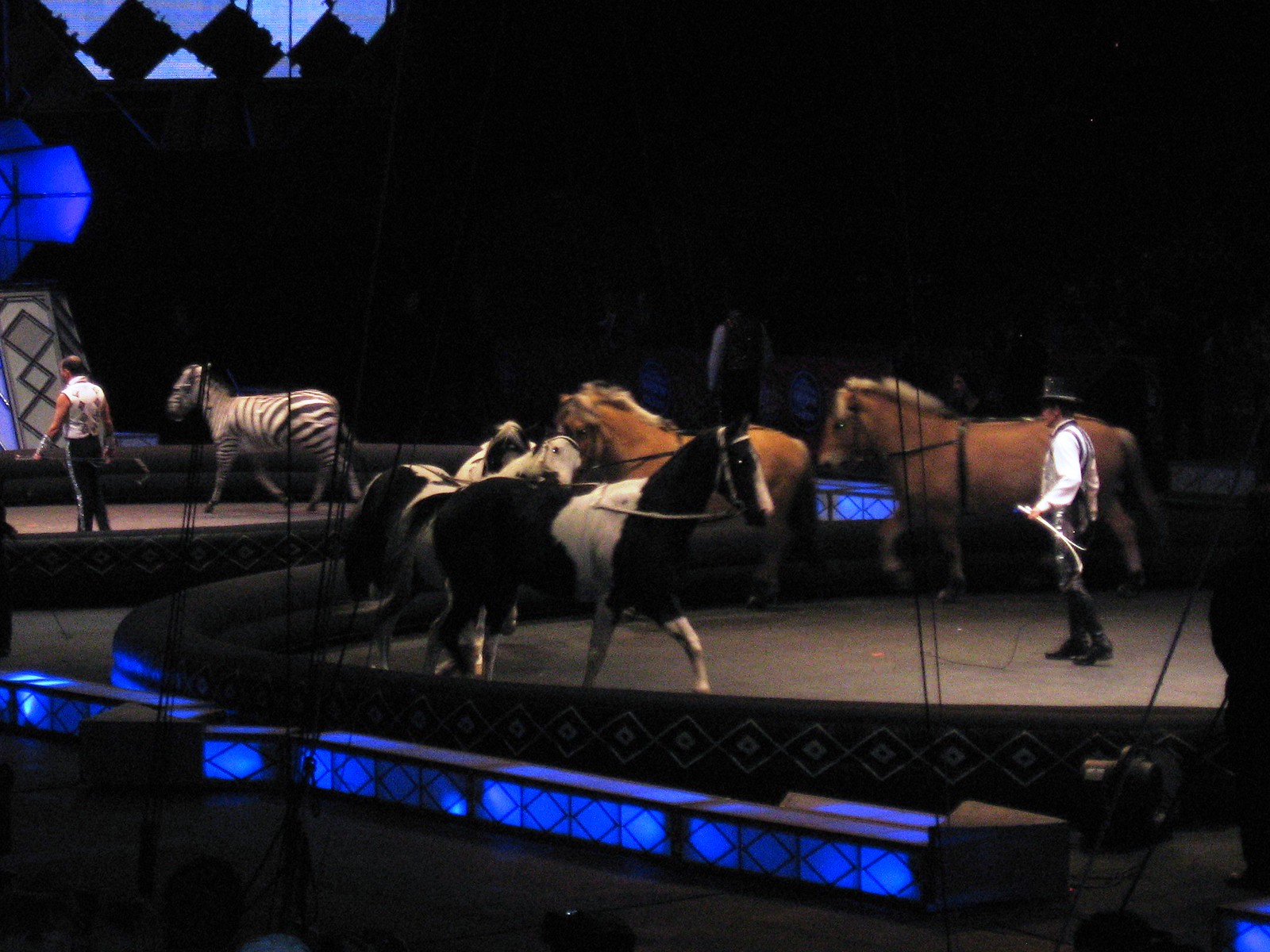The image captures a vibrant three-ring circus scene under blue ambient lighting, featuring a variety of horses and a potential zebra. In the center ring, dominated by a well-lit spotlight, five horses—two brown and three black and white paints—trot in a circle under the guidance of a traditionally dressed ringmaster. This ringmaster, wearing quintessential circus attire including black pants, a white shirt, a vest, and a hat, holds a whip, adding a theatrical flourish to the scene.

To the left, an intriguing sight unfolds as a similarly dressed trainer, accentuated by a vest with red diamond patterns and black wristbands, directs what appears to be a zebra. This might provoke curiosity about whether it's a genuine zebra or a painted horse. Both rings are adorned with low walls featuring diamond designs, illuminated blue lighting running across their bases and emanating from above, casting a mystical glow.

The background offers a stark contrast with its ominous black, drawing more focus to the illuminated spectacles in the rings. Hints of a seated audience barely emerge from the darkness, emphasizing the performers and their surrounded enclosures. The overall portrayal captures the essence of a traditional circus intertwined with modern lighting aesthetics, showcasing the elaborate display of animal acts, though it subtly nods to the ethical complexities behind such performances.